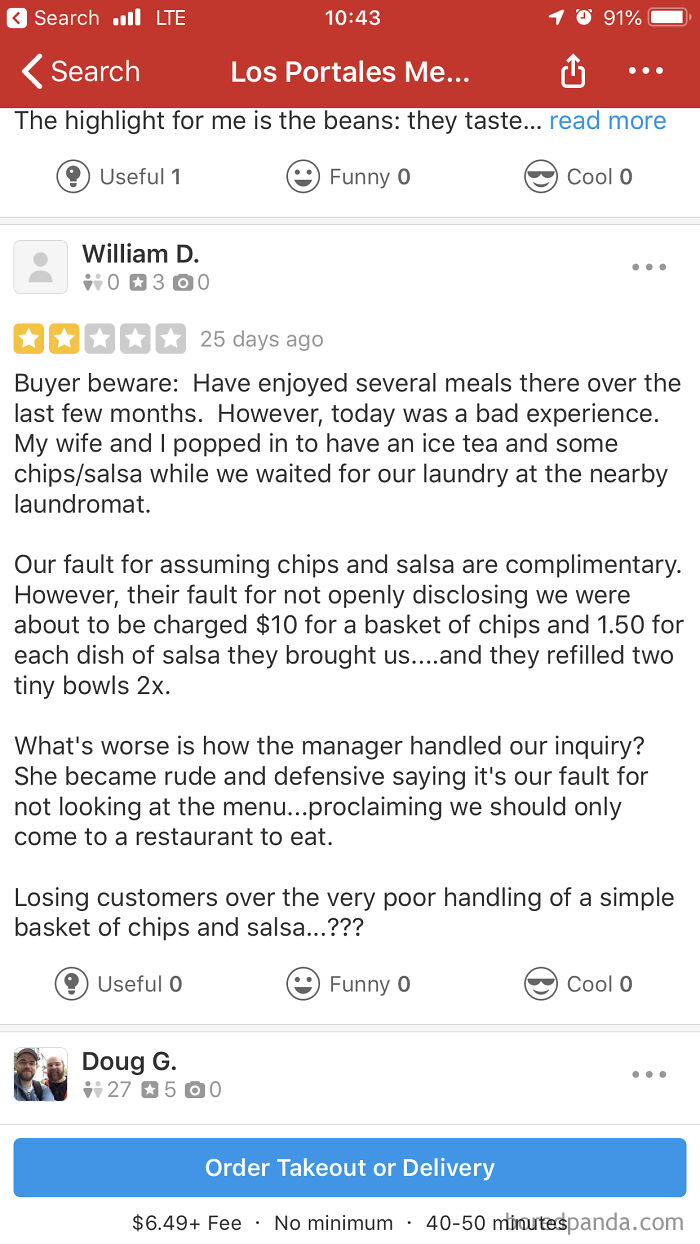This image is a vertical screenshot taken from a cell phone. At the very top, there's a red header featuring a search bar with an arrow pointing to the left. The text "Los Portales ME" is displayed next to three horizontal dots, indicating a menu option.

Beneath the header lies a review section. The first visible review begins with the line, "The highlight for me is the beans: they taste... read more," in black text, followed by a blue "read more" link. 

Directly below, a review by "William D" is prominently featured. His review has an avatar placeholder image, indicating the absence of a personal photo. He rated the restaurant 2 out of 5 stars and titled his review "Buyer Beware." 

The review details a disappointing experience where William and his wife visited the restaurant to enjoy iced tea and chips with salsa while waiting for their laundry at a nearby laundromat. They were surprised by the charges: $10 for a basket of chips and $1.50 for each salsa serving, despite receiving two refills of the tiny bowls. William critiques the management's response when he inquired about the charges, noting that the manager became rude and defensive, blaming the couple for not checking the menu and suggesting that they should visit the restaurant only for dining purposes. William questions the rationale behind potentially losing customers over mishandling such a minor issue.

A subsequent review by "Doug G" is partially visible, accompanied by an image of a couple on the left.

At the bottom of the screen, there is a prominent blue bar with the options to "Order Takeout or Delivery," suggesting that this screenshot is from the restaurant's website where users can review and order. William's review is notably critical, reflecting his dissatisfaction with the establishment.